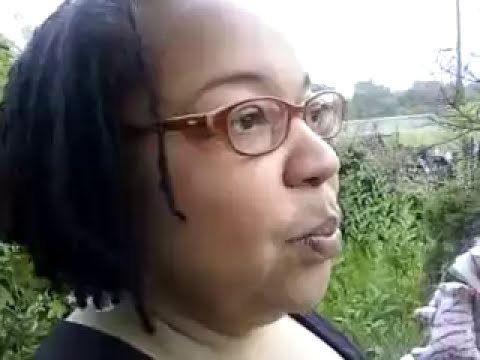The image is a color photograph taken outdoors during the daytime, focusing on a heavyset, younger African-American woman with a light caramel complexion. Her dark black hair appears to be styled in short braids, dreadlocks, or cornrows, though the picture is somewhat blurry. She is wearing brown-framed glasses with clear lenses and a dark-colored top with a lower cut scoop neckline. Her face is neutral, with her brown eyes looking intently to the right. The background features various greenery, including bushes, plants, and possibly some tall grasses or leaves, as well as a vertical branch or trunk in the top right corner. The sky is cloudy or washed out by bright sunlight, making the scene appear somewhat dull. There is also a grayish rock formation in the bottom right of the image. The entire image is slightly hazy and out of focus, suggesting it might be a still from a low-quality video or a zoomed-in portion of a larger picture.